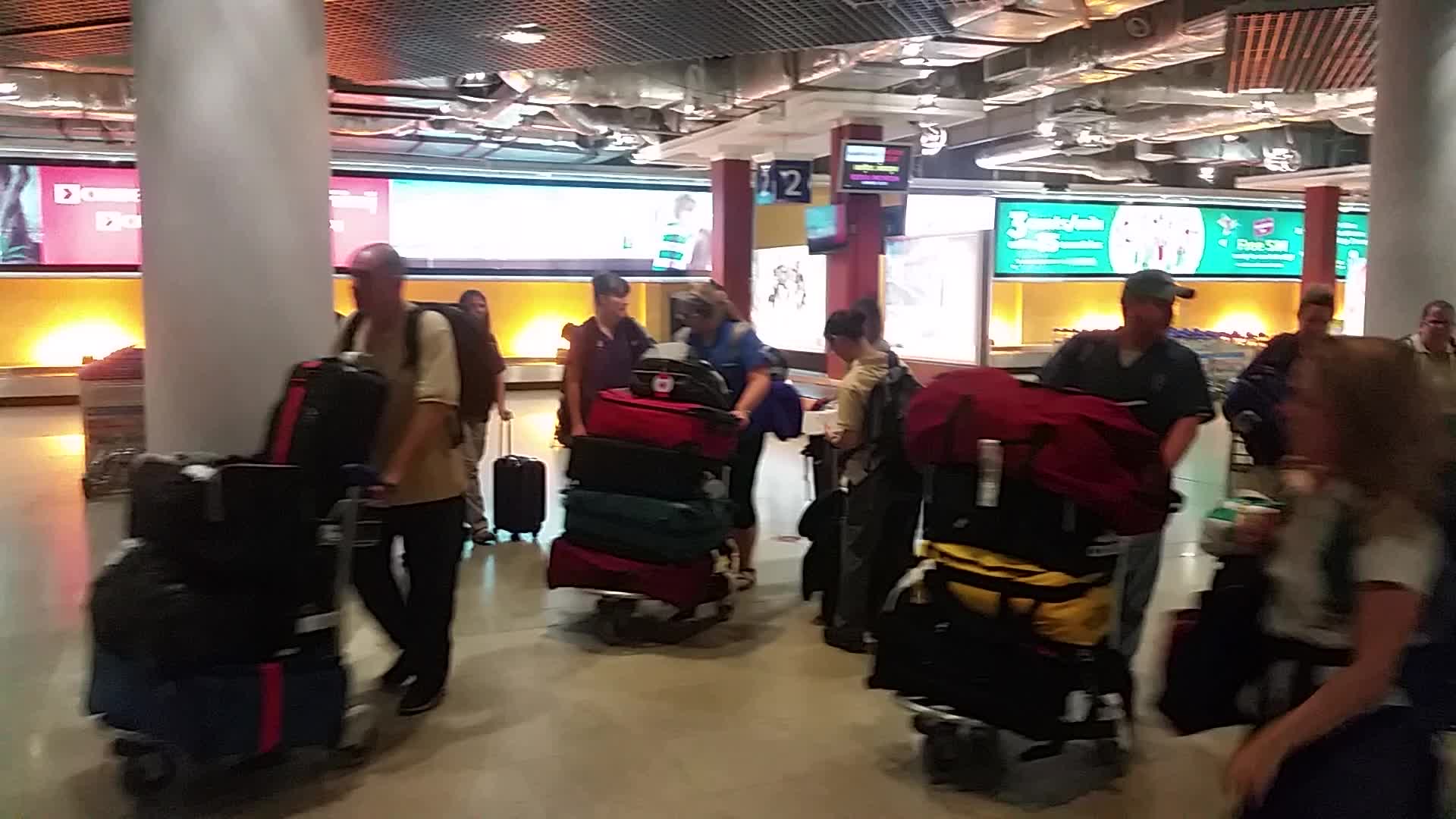In this dimly lit, blurry, amateur photo captured inside an airport terminal at the baggage checkout, a group of people is shown retrieving their bags from the roundabout baggage collection area, identified by the visible number 2. The individuals are pushing wheeled luggage carts, with some carrying suitcases stacked in buggies and others pulling single suitcases. The photo is crowded with at least nine people, none of whom are looking at the camera, making their faces indiscernible. The background features indistinct advertisements on large lit-up boards and signs, along with notable architectural elements such as two huge beige cylindrical posts supporting the ceiling and some red to black posts. Among the luggage, one bag prominently displays a Canadian flag. The overall quality is poor, with motion blur adding to the indistinctness.